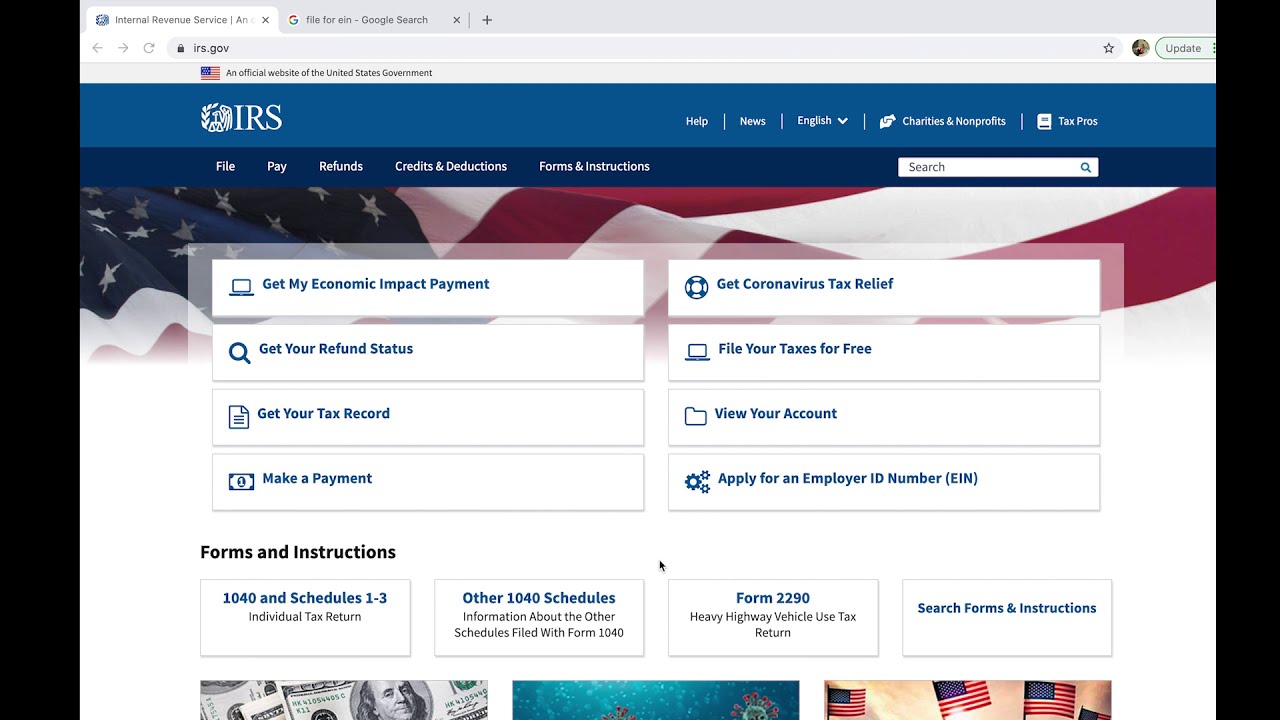This screenshot captures the homepage of the IRS website, IRS.gov, labeled as an official website of the United States government. The layout begins with a medium blue header displaying the IRS logo and the word "IRS," followed by navigational tabs with options like Help, News, English, Charities & Nonprofits, and Tax Pros. Below, a darker navigation bar provides additional choices: File, Pay, Refunds, Credits & Deductions, and Forms & Instructions, alongside a search text box with a magnifying glass icon.

The middle section of the page features an American flag as the backdrop, transitioning to a plain white lower half. Central to this area are eight informative rectangles, each with a title and icon. They are organized as follows:
1. Get My Economic Impact Payment
2. Get Coronavirus Tax Relief
3. Get Your Refund Status
4. File Your Taxes For Free
5. Get Your Tax Record
6. View Your Account
7. Make a Payment
8. Apply for an Employer ID Number (EIN)

A subheading labeled "Forms and Instructions" introduces further resources:
- 1040 and Schedules 1-3 for Individual Tax Returns
- Other 1040 Schedules, providing details on additional forms filed with Form 1040
- Form 2290, Heavy Highway Vehicle Use Tax Return

The section concludes with a final heading for "Search Forms and Instructions."

At the bottom of the page, the footer displays partial images that include a dollar bill, a coronavirus illustration, and a graphic featuring three American flags.